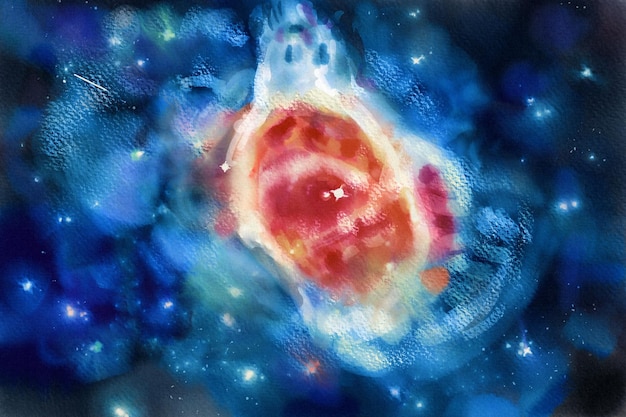The image appears to be a highly abstract and artistic depiction, likely created using digital or traditional painting techniques. Its overall mood is dark and enigmatic, dominated by deep navy blue and black hues, evoking the vastness of space. The composition features a central luminous area with a core of intense red that gradually transitions through shades of orange and yellow, finally bordered by an off-white glow. Surrounding this vibrant core are hazy areas of light blue, blending seamlessly with the darker background, reminiscent of a nebula or galactic phenomenon.

The texture of the image suggests a medium such as watercolor, oil painting, or even chalk, as nothing in the image is crisply defined; rather, everything softly blurs together. This effect enhances its ethereal, cosmic feel. Scattered throughout the image are small white dots, mimicking stars scattered across a celestial landscape. With around twenty stars clustered around the central area and a particularly bright star at the center, the scene draws immediate attention to its vivid, almost explosive core, evoking the imagery of a supernova.

Overall, the abstract nature and the blending of vivid and dark colors with scattered star-like dots create an impression of a galactic or nebulous scene, inviting the viewer to ponder its cosmic beauty.